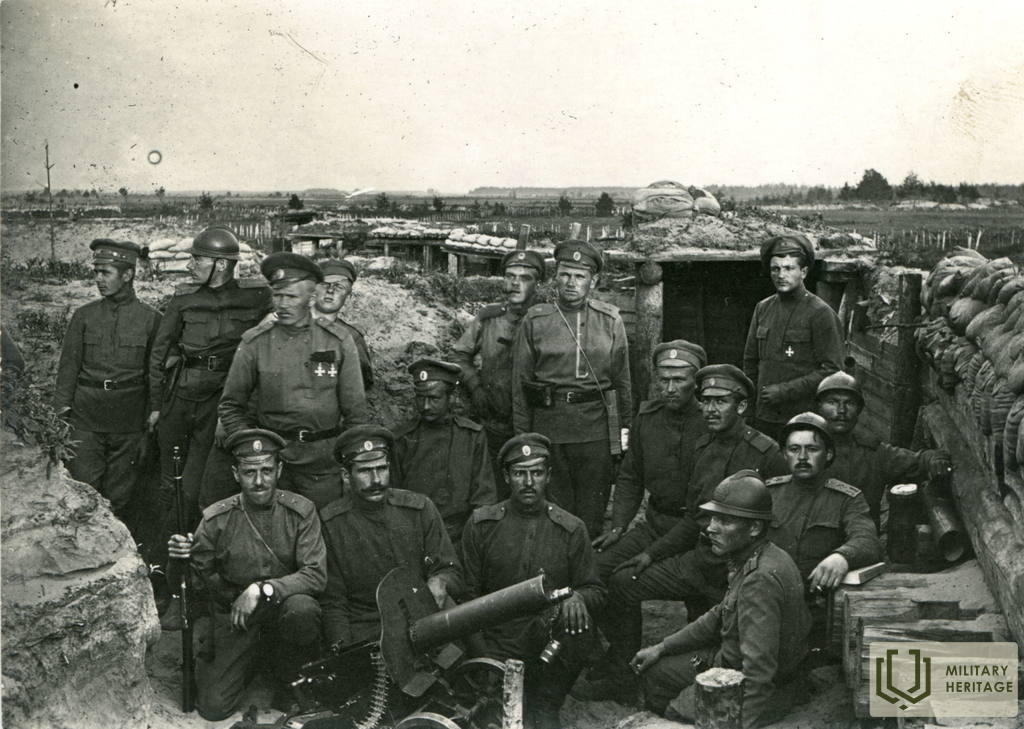This black-and-white photograph, likely from World War I, depicts a group of about 19-20 soldiers in a trench. They are predominantly wearing uniforms with either berets, hats, or helmets. The men are situated in and around a dug-out bunker camouflaged into a hillside, with its open doors revealing the interior. At the front of the group is a small cannon, possibly a Vickers machine gun, while several soldiers hold rifles. Most soldiers are looking directly into the camera, with a few scanning the surroundings, potentially for approaching enemies. The setting is rugged, featuring mostly dirt, rocks, and some scattered trees, with a wide, open field and larger trees seen in the background. A box in the lower right of the image is labeled "Military Heritage," reinforcing the historical significance of the scene.